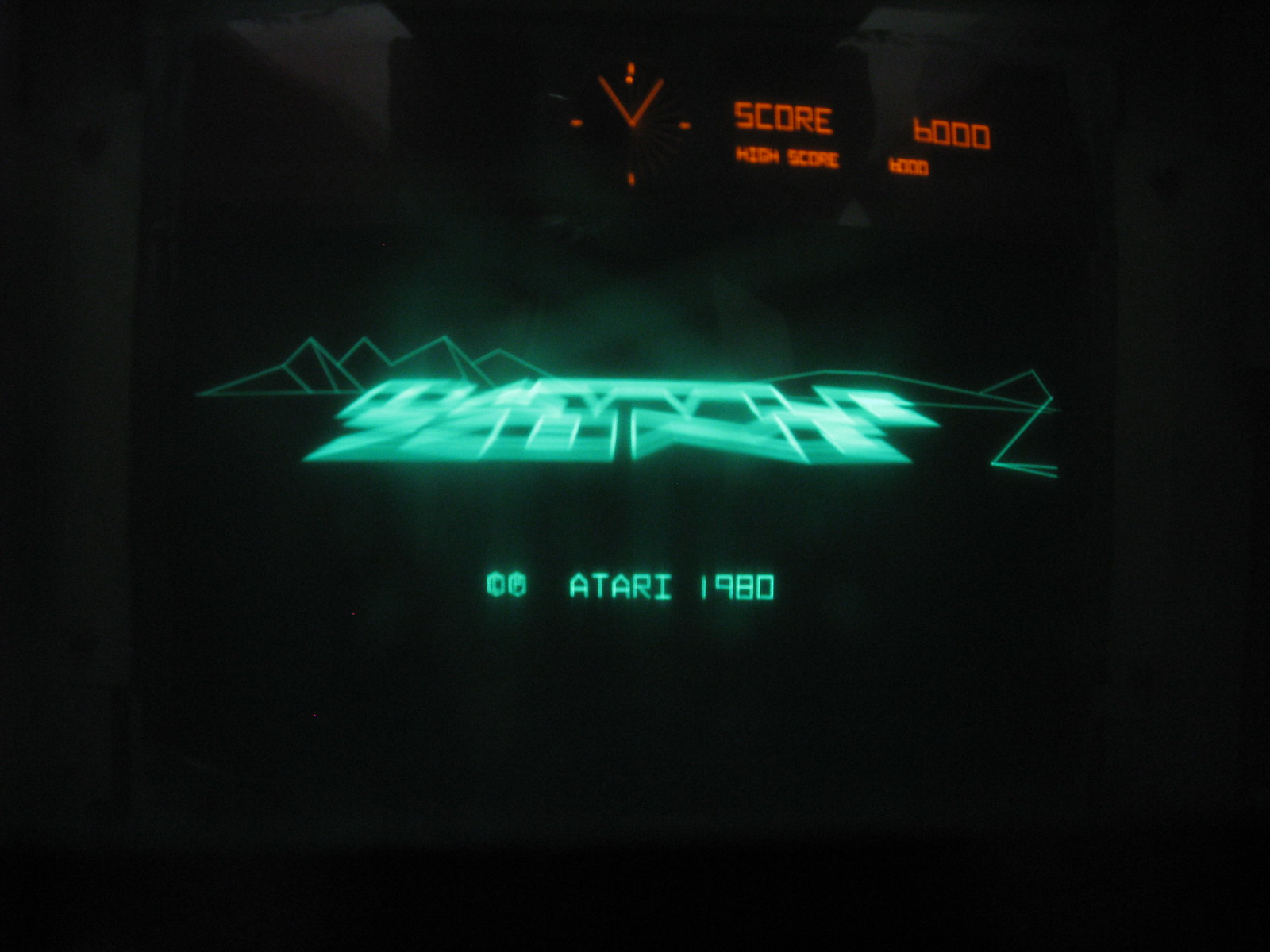In the detailed view of this vintage video game screen, the predominant color is black, with slight reflections visible off its glass surface. Dominating the screen is a horizontal, icy blue lettering that vaguely reads "Zotor," situated right above a series of crudely drawn, angular mountains in a matching hue. Just below this, the text "Atari 1980" is displayed in the same blue, accompanied by two small diamond symbols to its right. Above this text is a section of illuminated orange letters, partially out of view. To the left of the orange text, an analog clock face shows the time as ten minutes to one, marked only by hash marks to indicate the hours, devoid of numerical indicators. To the right of this clock, the word "SCORE" appears in capital letters, followed by the number "6000." Beneath this, the words "HIGH SCORE" are also followed by "6000," indicating that this score is potentially the highest achieved in the game so far. This setup, complete with the rugged aesthetics and nostalgic design elements, suggests the device is likely a console in a classic video game arcade.